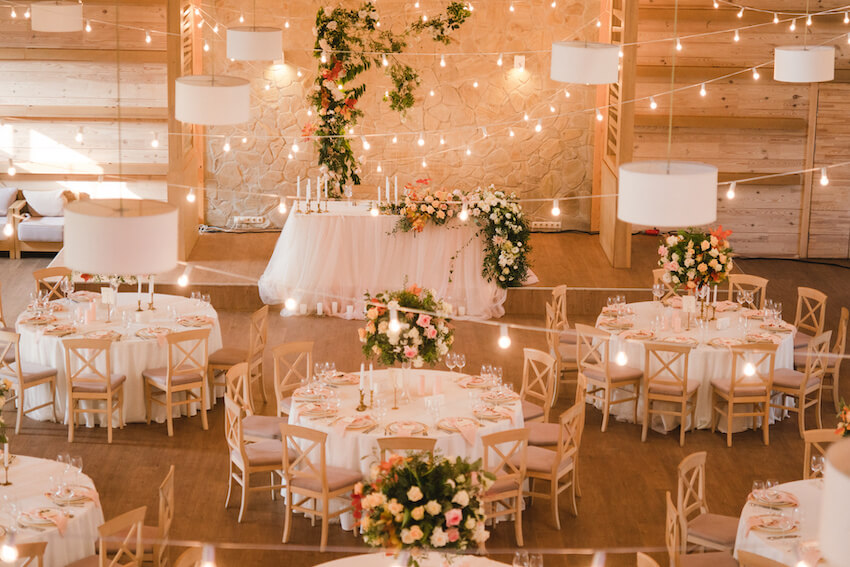The image captures an elegantly decorated reception hall, likely set up for a wedding. It is a full-color, square photograph taken from an elevated perspective, looking down at the indoor venue illuminated by artificial light. The hall features a wooden floor and is adorned with numerous round tables covered in pristine white tablecloths. Each table is surrounded by wooden chairs with white cushions and showcases a large floral arrangement composed of roses in shades of yellow, pink, and white, intertwined with lush greenery.

Strung across the ceiling, delicate strings of small white light bulbs create an enchanting star-like canopy, while larger white chandeliers add an extra touch of sophistication. In addition to the floral centerpieces, each table is embellished with wine glasses and clusters of candles, enhancing the intimate ambiance. The back wall is artistically decorated with garlands, framing an elongated head table intended for the bridal party. This table is ornately arranged with a mix of candles, an overflow of greenery, and additional flowers cascading gracefully off one side. The room is impeccably set up and waiting for guests to arrive, exuding a sense of serene elegance and festive expectation.